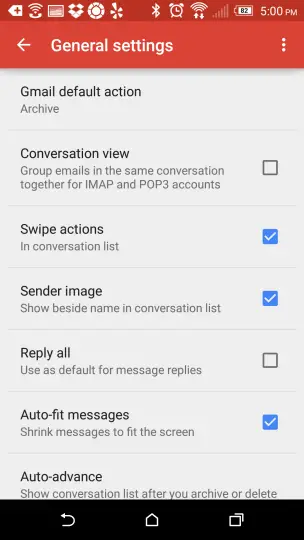A detailed and cleaned-up caption for the image could be:

---

The image is a screenshot of the "General Settings" tab in the Gmail app, captured on a mobile device, likely running Android. 

At the very top, the status bar displays several icons, including a Wi-Fi symbol, multiple app notifications, Bluetooth, a mobile data indicator, a clock showing 5:00 PM, and a battery icon.

Directly beneath the status bar, within a segment bar indicating the current section, a back button appears on the left, and the label "General settings" is centered.

The settings options listed from top to bottom are:

1. **Gmail default action:** Set to Archive.
2. **Conversation view:** This setting, which groups emails into conversations for IMAP and POP3 accounts, is unchecked.
3. **Swipe actions:** This setting, enabling swipe actions in the conversation list, is checked.
4. **Sender image:** This setting, showing the sender's image beside their name in the conversation list, is checked.
5. **Reply all:** The option to use "Reply all" as the default for message replies is unchecked.
6. **Auto fit messages:** The option to shrink messages to fit the screen is unchecked.
7. **Auto advance:** The partially visible description suggests that this setting allows the conversation list to be shown after archiving or deleting messages.

At the bottom of the screen, the navigation bar shows three icons: a back button, a home button, and a recent apps button, characteristic of an Android device.

---